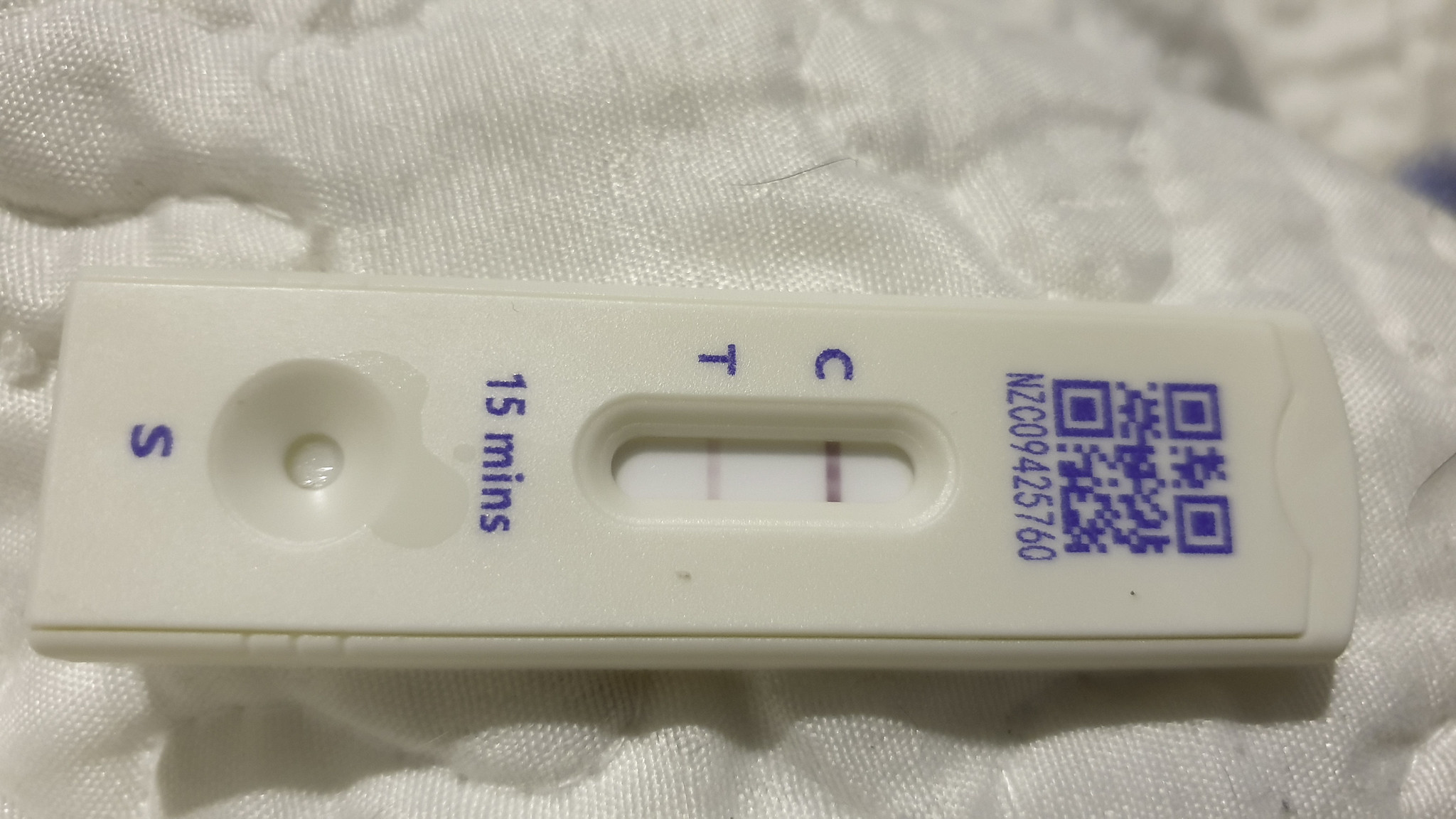The image captures a white plastic COVID-19 test positioned horizontally on a billowy, fluffy piece of styrofoam, which is intricately grooved with dark gray lines defining its depressions. The porous, foam-like texture of the styrofoam adds a dynamic background to the scene. The COVID-19 test, with its bottom on the left side and top on the right, features a blue QR code on a white background at its top end. Directly beneath the QR code is a clear oval window bordered by dark blue letters "C" and "T", serving as markers for the test results. Below this window is an indication of "15 minutes" in blue text, providing a time reference for the test. Further down, there's a well intended for the liquid sample, which appears slightly depressed and moist, casting a shadowy edge at its center. The well is marked by a blue letter "S" situated centrally on the left-hand side of the test.